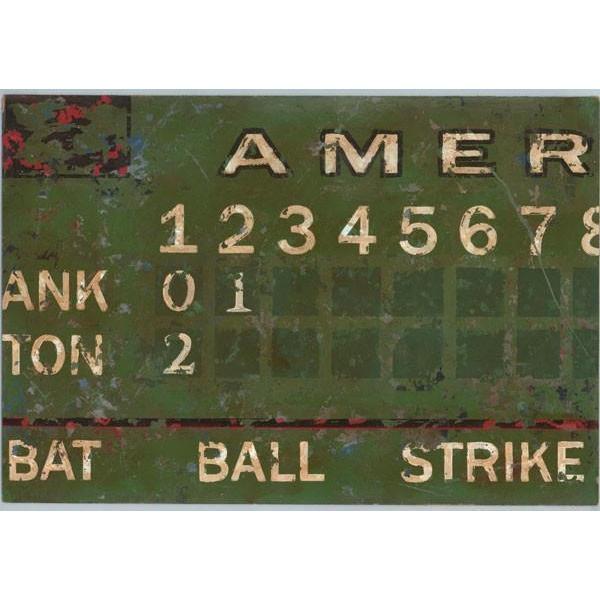This image is a detailed close-up of an old-fashioned, weathered baseball scoreboard, which appears almost like a piece of artwork due to its condition and age. The main color of the scoreboard is a dark, forest green, with texture and chips that expose layers of light blue and red paint underneath. At the top, in bone white text with a black outline, the letters "AMER" are visible. Below this, the numbers 1 through 8 are displayed, also in bone white. Under these numbers, green squares display scores, including a 0 under the first column and a 1 under the second. Additionally, there are the indistinct names "ANK" and something resembling "NON" or "TON." The lower section of the scoreboard features worn text for "bat," "ball," and "strike." The entire sign is nicked and the paint is chipping, giving it an appearance as though it has been submerged in water or left to weather for decades.